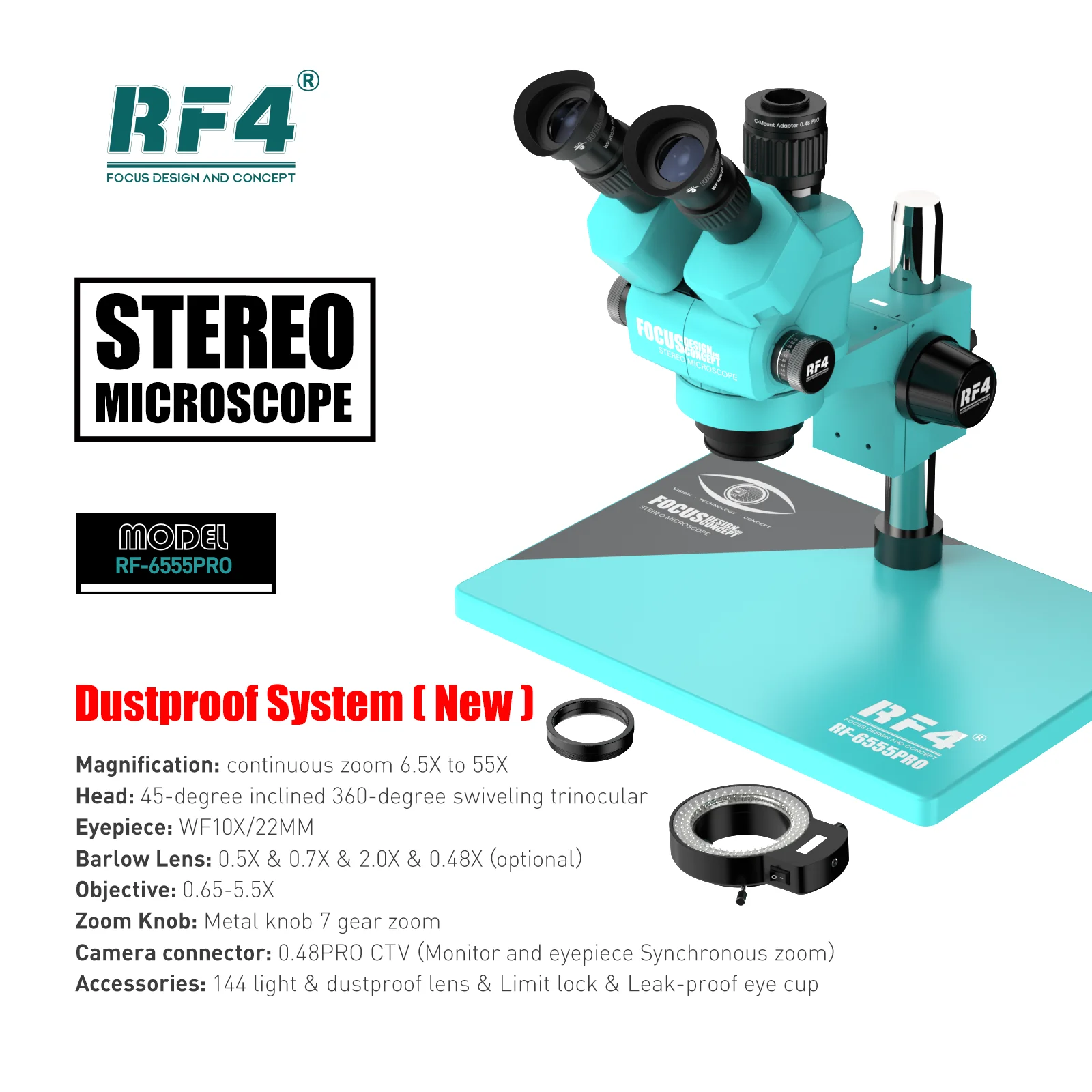The image is an advertisement for a stereo microscope, specifically the RF-6555 Pro model. The advertisement features detailed specifications prominently displayed in a black rectangular box with white outlined text. These specs cover various aspects such as the dustproof system, continuous zoom magnification ranging from 6.5x to 55x, a 45-degree inclined trinocular head with a 360-degree swivel, and WF-10x 22 mm eyepieces with a Barlow lens. The specs text includes elements in bold black font and non-bolded text, providing clear and detailed information.

The microscope itself is a striking robin's egg blue and is mounted on a large rectangular platform base. The image includes a watermark in the top left corner that states "RF-4 focus and design concept." The knobs used for adjusting the microscope are black and feature the RF-4 logo. Additional text in the image highlights key features such as "dustproof system" in red Impact font and the term "stereo microscope" also in Impact font, designed with black text on a white rectangular background with a black border.